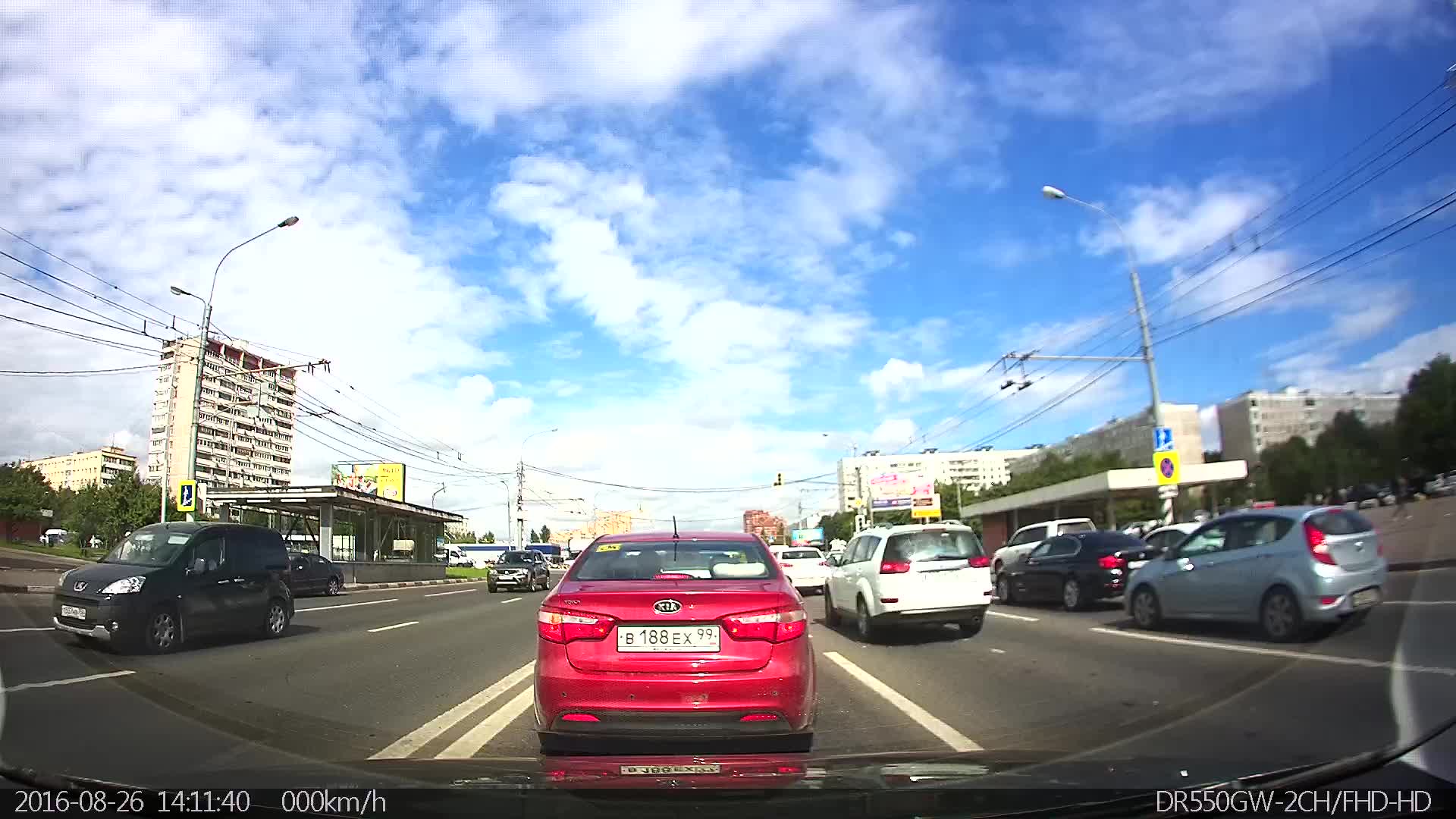The image depicts a bustling city street scene captured from a dashcam on August 26th, 2016, at 1411 hours and 40 seconds. The foreground is dominated by the tail end of a red Kia, easily identifiable by its long rectangular white tag with black writing. This car is positioned in a lane adjacent to two solid lines. The street, made of asphalt, accommodates six lanes of traffic with various cars moving in both directions, divided by solid and dotted white lines. Notably, the next lane features a white car, followed by a blue car, and one lane remains momentarily unoccupied. The city's skyline frames this urban tableau, with several high-rise buildings, including a prominent white skyscraper adorned with numerous windows, flanking the road. Commercial buildings, tall streetlights, telephone lines, and power lines stretch along the roadway. The brilliant blue sky above is scattered with variegated clouds, adding a dynamic backdrop to the bustling traffic scene. The bottom right corner of the image includes a digital timestamp and a code: DR 55 OGW / 2CH / FHD / HD, likely indicative of its origin from a surveillance or dash camera.